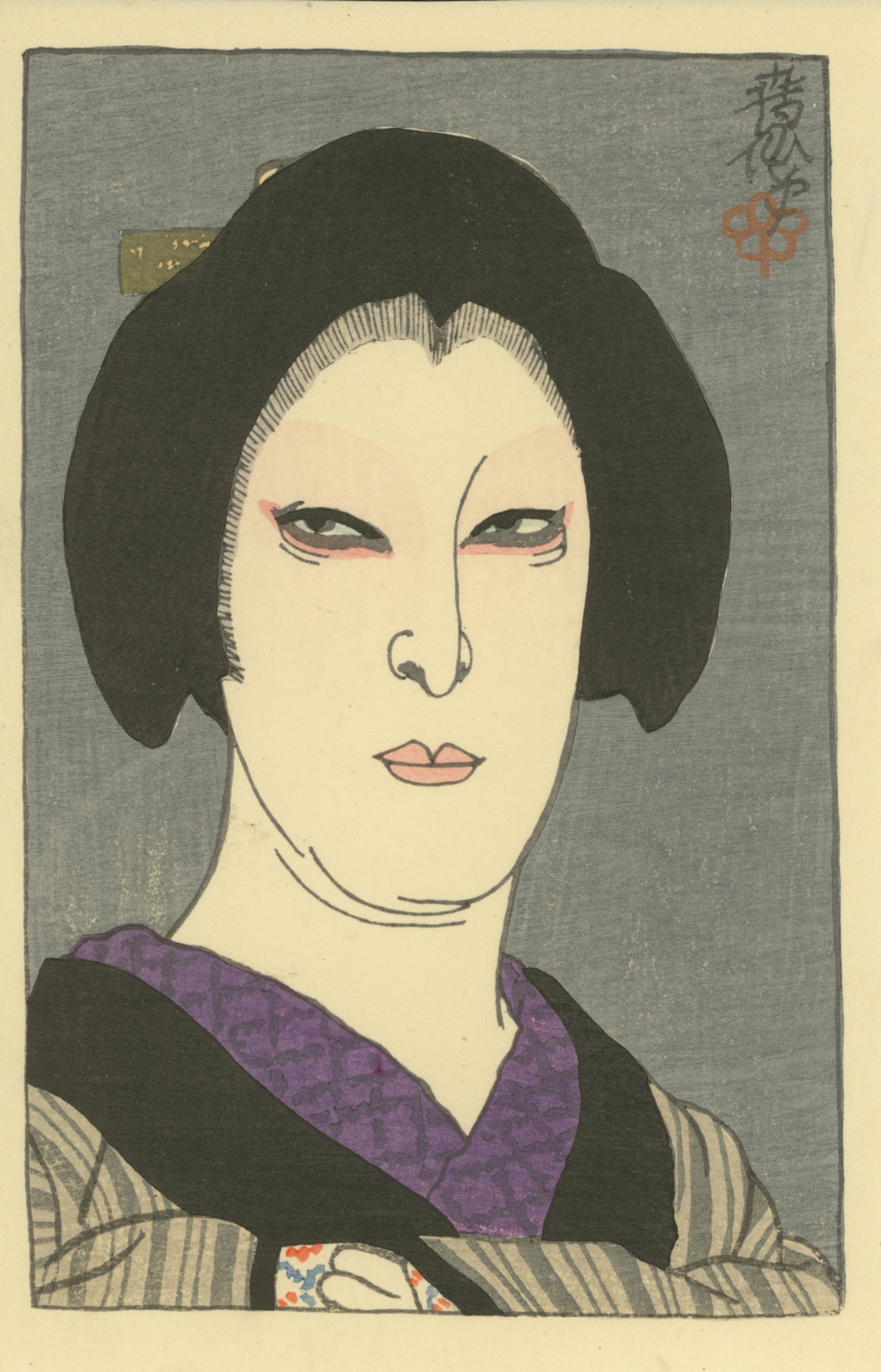The image is a detailed and evocative watercolor portrait, possibly mixed with pen or ink, featuring an Asian woman with a serious and solemn expression. She has striking black hair styled into a traditional headpiece that comes down to her ears, forming a widow’s peak at the forehead. Her eyes are thin and surrounded by gray and peach highlights, which give them a tired and intense appearance, further accentuated by pinkish coloring beneath them. Her lips are a soft pinkish peach.

The woman is draped in a traditional kimono with a complex layering of colors and patterns: an inner part with a purple diamond pattern, a black lapel, and an outer layer featuring vertical gray and white stripes. Her sleeves are adorned with orange and blue flower prints. In the upper right corner of the image, there is an inscription in what appears to be Japanese or Chinese characters, accompanied by a small red flower.

The composition is set against a muted, dark gray background, framed by a thin beige border that highlights the central figure. The intricate details and the interplay of colors and textures contribute to the somber yet mesmerizing quality of the portrait, evoking a sense of traditional Asian artistry and cultural depth.